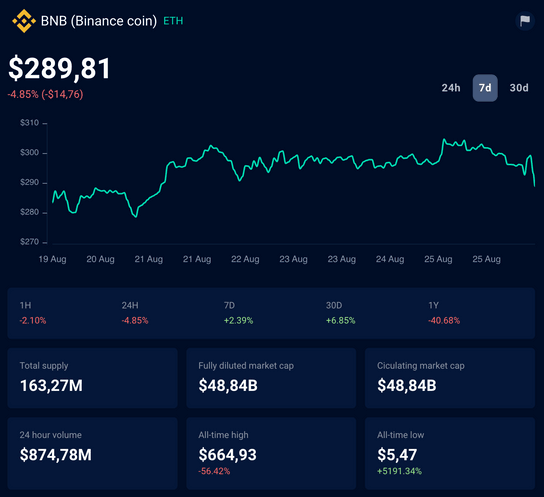The image is a screenshot of a cryptocurrency trading platform, likely Robinhood, displaying detailed information about Binance Coin (BNB). The background is predominantly black with bluish-black information boxes, creating a sharp contrast that highlights the displayed data. 

At the top of the screenshot, a small yellow diamond-shaped logo is present alongside the label "BNB," referencing Binance Coin, and "ETH" in green, suggesting a comparison or related information with Ethereum. The current price of Binance Coin is shown as $289.81, accompanied by a red indicator showing a decrease of 4.85% or $14.76.

An option bar allows the user to switch between views of data over different time periods: 24 hours, 7 days, and 30 days. A graph beneath this option bar illustrates the fluctuating price of Binance Coin with a wavy green line. Dates are marked along the bottom of the graph, while the vertical axis on the left shows price points.

Below the graph, the screenshot features additional information boxes in a bluish-black hue. The top section appears to summarize the change in the stock price over the selected time periods. The lower section consists of six boxes arranged in two rows of three, displaying various metrics such as "Total Supply" and "Fully Diluted Market Cap," providing further insights into Binance Coin's trading data.